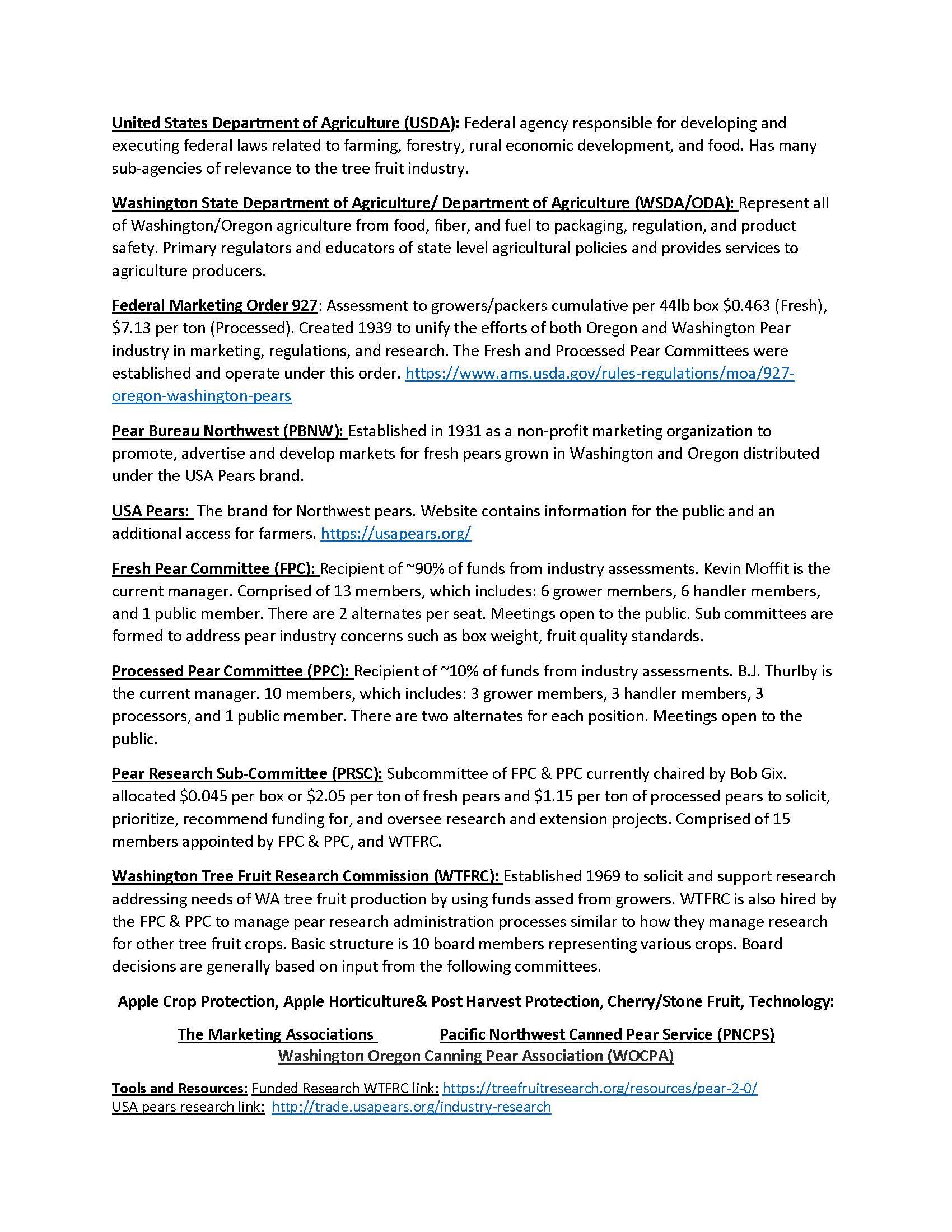**United States Department of Agriculture (USDA): A Comprehensive Overview** 

The image features a white background prominently displaying the bolded text "United States Department of Agriculture (USDA)." This title introduces the USDA as a federal agency responsible for developing and executing federal laws related to farming, forestry, rural economic development, and food. Various sub-agencies of particular relevance to the tree fruit industry are mentioned.

**Washington State Department of Agriculture (WSDA/DDA):**

The next section highlights the Washington State Department of Agriculture, denoted as WSDA/DDA. 

**Federal Marketing Order 927:**

This segment provides information about Federal Marketing Order 927 and several pertinent details, concluding with a blue hyperlink for additional resources.

**Pears and Related Information:**

Following this, information about pears is presented, including specific categories such as "pear," "burro," "northwest," and abbreviations like "P," "B," "N," and "W." The section also includes a link to USA Pears information, designated by a blue hyperlink.

**Committees and Their Roles:**

The final segments introduce various committees related to pear farming:

- **Fresh Pear Committee (FPC):** Accompanied by relevant details.
- **Processed Pear Committee (PPC):** Includes pertinent information.
- **Pear Research Subcommittee (PRSC):** Also supplemented with related information.

Each committee’s section provides detailed descriptions of its roles and responsibilities within the pear industry. 

Overall, the image acts as an informative guide to the USDA and its sub-agencies, specifically focusing on their impact on the tree fruit industry, with an emphasis on pears.